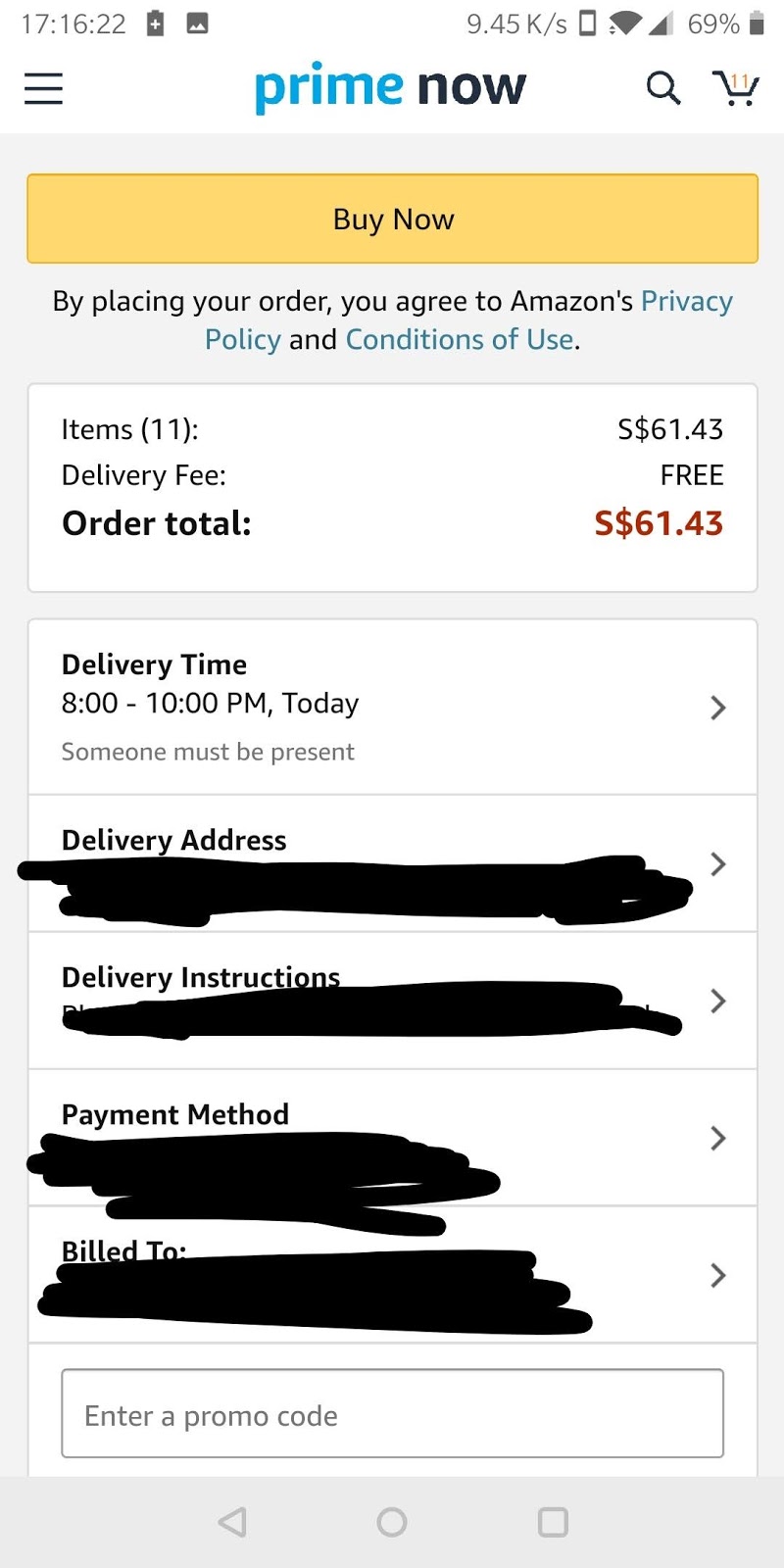This screenshot captures a detailed view of the Amazon Prime Now app on a smartphone. The top left corner prominently displays the current time and battery status. The app's header showcases the "Prime Now" logo with "Prime" in blue and "Now" in black, accompanied by a menu icon consisting of three horizontal lines. To the right, there is a search icon, a shopping cart displaying the number "11," indicating the quantity of items, and a yellow "Buy Now" button prominently positioned below these elements.

The screen further details the purchasing options: "By placing your order, you agree to Amazon's privacy policy and conditions of use." The section summarizes the order with the label "Items (11)," a subtotal of "$61.43," and confirms a "Delivery fee: Free." The total order amount is highlighted in red, "$61.43," with an expected delivery time between 8 to 10 p.m. today, noting that someone must be present to receive the delivery.

Four sections, labeled "Delivery address," "Delivery instructions," "Payment method," and "Bill to," each feature a right arrow for further details but have been blacked out, likely for privacy reasons. At the bottom of the screen, there is an input field for "Enter a promo code," followed by navigation icons: a back arrow, a home button, and a square icon.

Overall, this image is a comprehensive representation of the checkout page on the Amazon Prime Now app, illustrating various details and interactive elements essential for completing an online purchase.